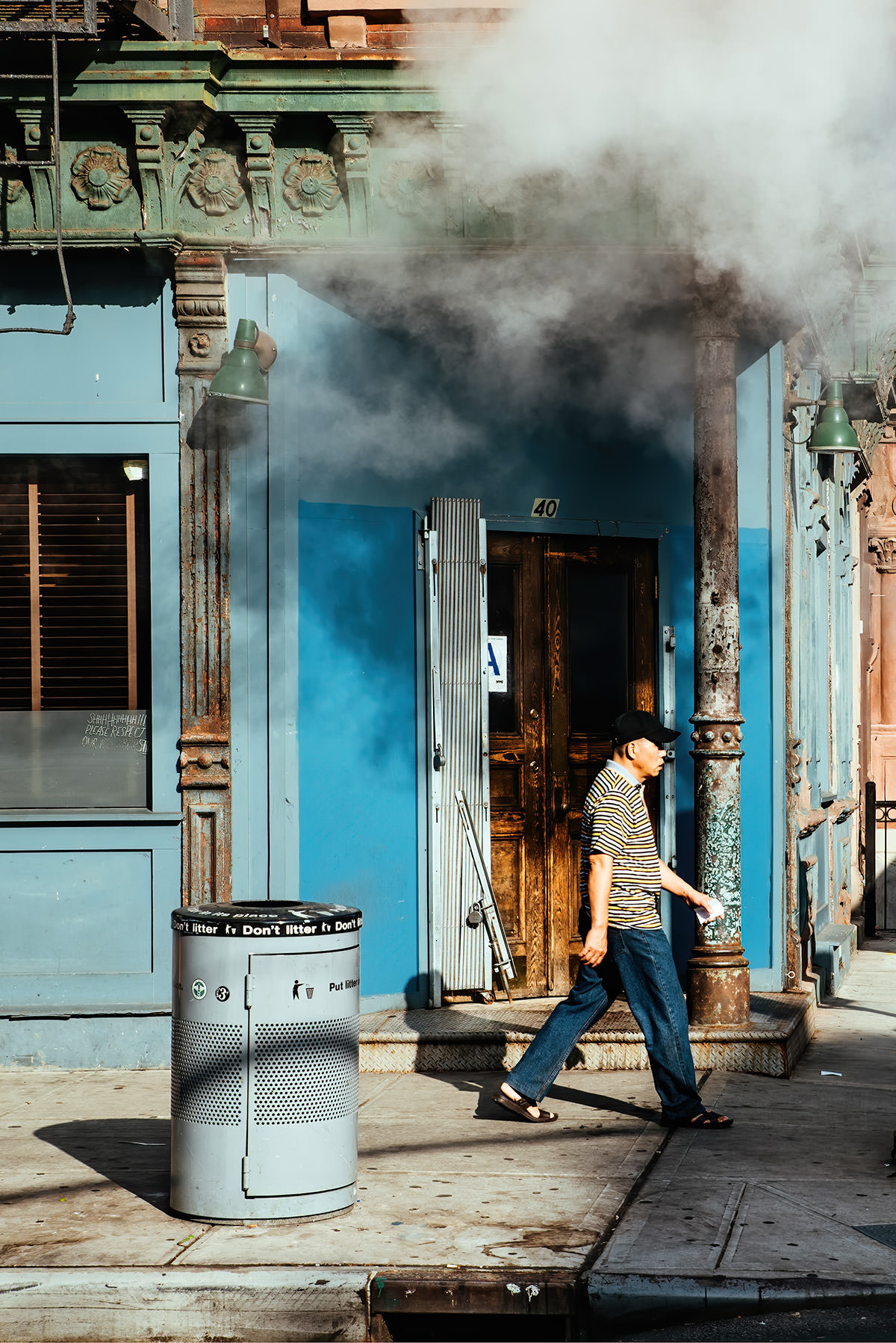In the image, a man is casually strolling down a cement concrete sidewalk, seemingly oblivious to the commotion around him. He's dressed in blue jeans, a black baseball cap, leather sandals, and a short-sleeve polo shirt with blue, brown, and yellow stripes. To his left, there's a large cylindrical, silver-gray garbage can with a black lid that prominently displays a "don't litter" sign alongside an illustration of someone properly disposing of trash.

A blue building with wooden double doors, partially obscured by an open metal gate, catches attention behind him. The building has a distinctive letter grade sign displayed in the window, indicating it may be a restaurant, a practice often seen in New York City. Above the door, the number '40' is visible. However, what truly stands out is the thick, billowing smoke escaping from the top of the building, a mix of dark gray and lighter white hues, suggesting a potential fire or intense cooking activity. Despite the concerning scene, the man appears unconcerned as he continues his leisurely walk, adding to the intriguing nature of the photo.